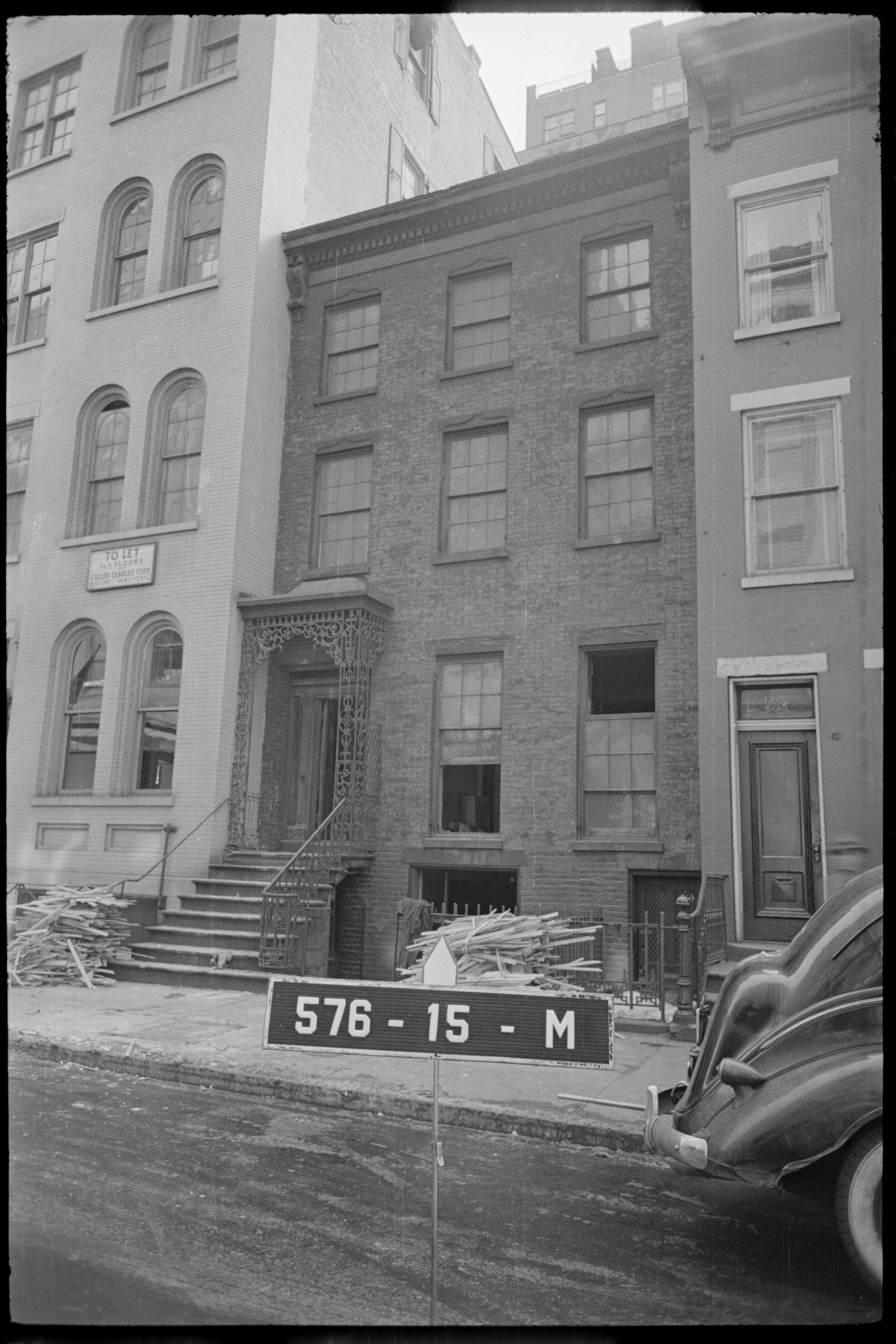This black and white photograph captures a historic urban street scene, featuring a prominent multi-level brick building at the center. The brick building, likely a refurbished brownstone from the 1940s, stands out with its architectural details, including a gabled porch and a mixture of windows and doors across its four levels, which include a basement, ground floor, first floor, and second floor. The top two floors each have three windows, the ground floor has two windows flanking a central door, and the basement features an additional window alongside a door.

This brick building is the shortest of three structures closely connected along the street. To its left, a taller building looms, while to its right, another slightly taller building stands. Near the front of the scene, a street sign marked "576-15-N" or "576-15-M" (the exact lettering is indistinct) stands prominently. Adjacent to this sign, partially out of frame, is the rear end of what appears to be an old Volkswagen Bug. Scattered piles of wood are visible, hinting at ongoing renovations. The entire scene, enveloped in grey tones, evokes a mid-20th-century American urban atmosphere.